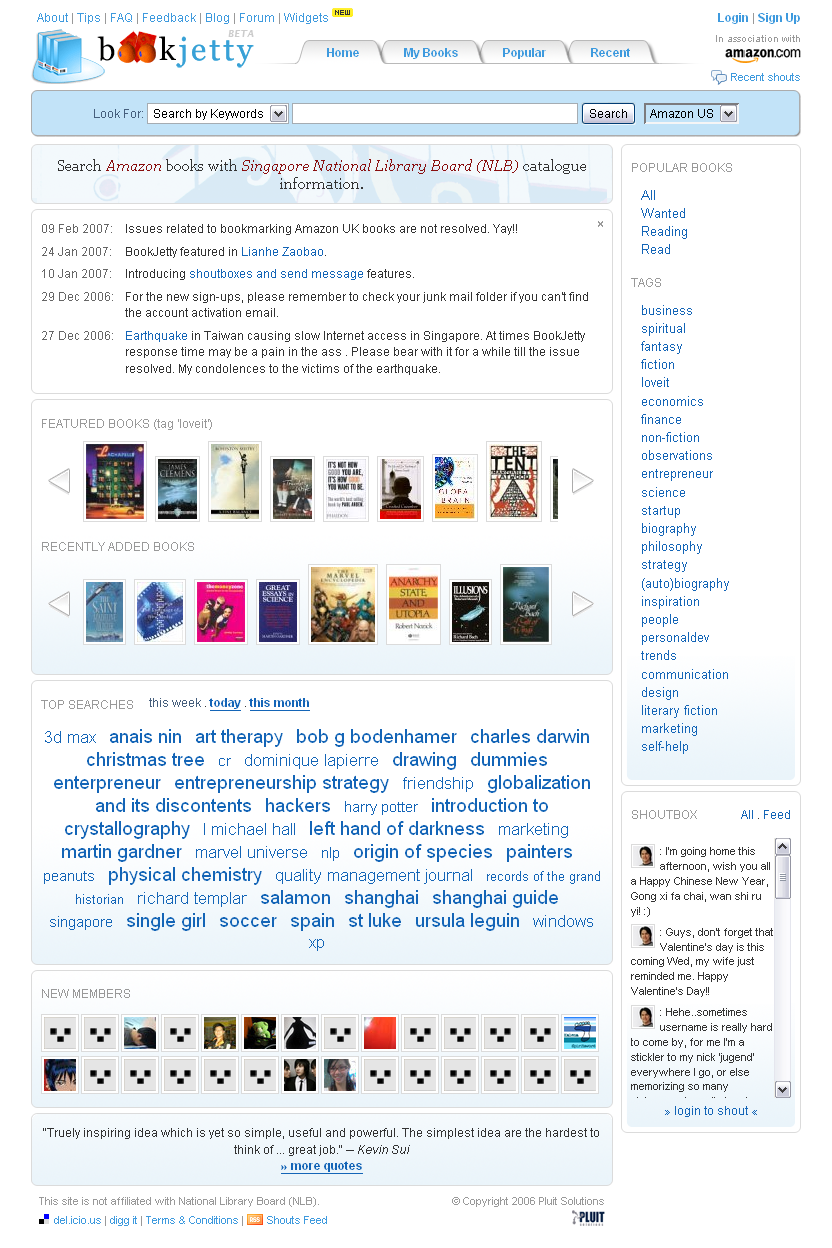A photo captures a computer screen displaying the homepage of "Book Jetty," likely accessible at bookjetty.com. The design of the logo creatively incorporates the word "BOOK" with the letters "B" and "K" in black font, while the two "O"s are styled to resemble oranges with blue dots, mimicking owl eyes. The word "JETTY" is written in blue, complementing the whimsical logo.

At the top navigation bar, key sections include "Home," "My Books," "Popular," and "Recent." Above this navigation bar, additional links such as "About," "Tips," "FAQs," "Feedback," "Blog," "Forum," and "Widgets" are displayed. A yellow banner with "New" inside highlights the "Widgets" option.

A noticeable red banner provides a search function with the text: "Search Amazon books with Singapore National Library Board Catalog, NLB." On the right-hand side of the screen, a section labeled "Popular Books" offers clickable options for categories like "All," "Wanted," "Reading," and "Read." Further down, there are various tags for additional navigation and exploration within the site.